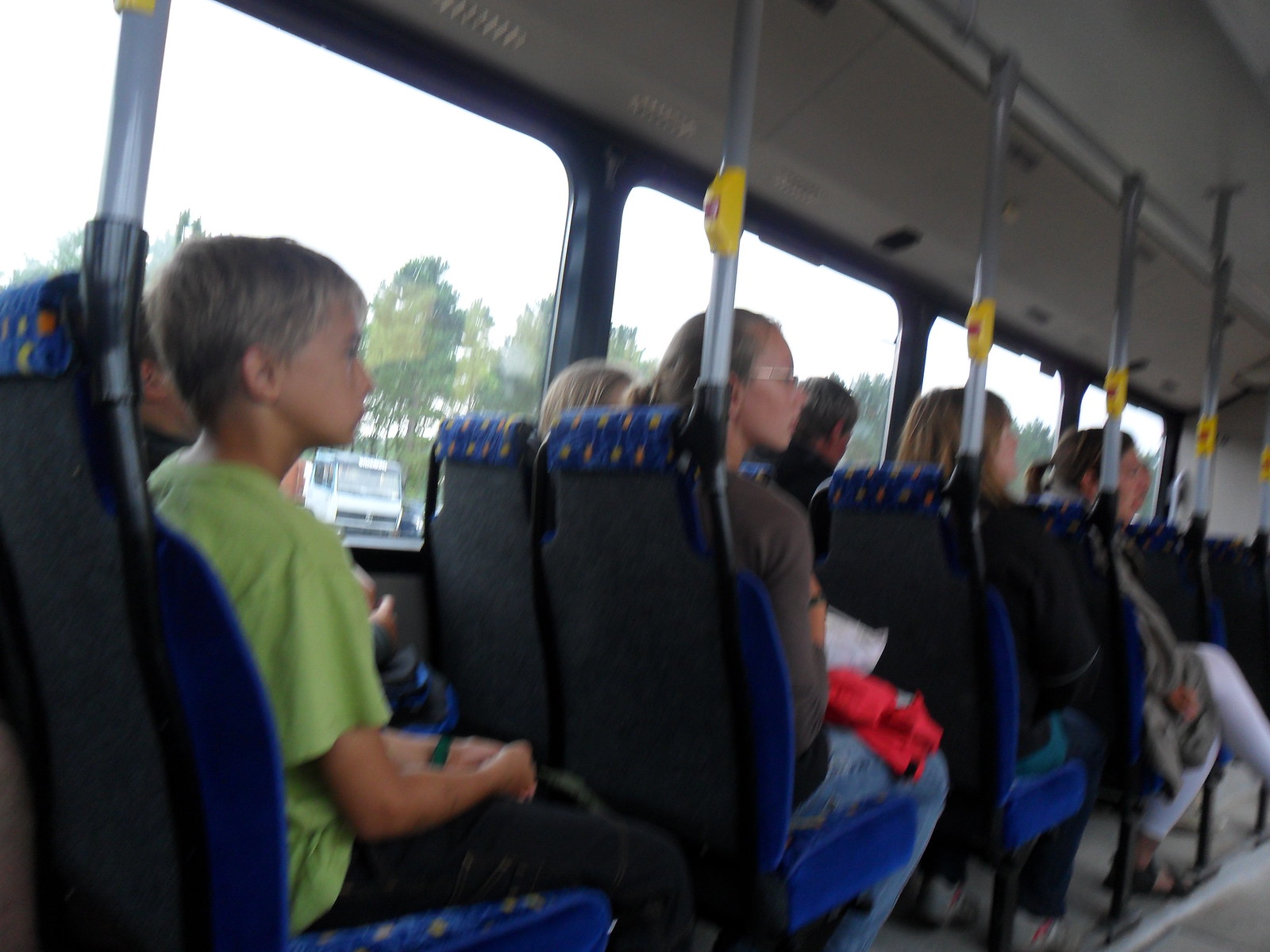The blurry photograph captures the inside of a seemingly upscale tour bus, filled predominantly with school-aged children and a few adults. Each seat features blue fabric upholstery with yellow and orange patterns, contrasted by hard black plastic seat backs. The seats are equipped with metal poles supporting yellow stop-request buttons. The children and young adults are seen casually dressed, with a notable young blonde boy in a green shirt and black pants seated toward the back, next to an indistinct figure. In front of him, a girl with glasses, brown hair pulled back, and a brown shirt with jeans holds a red item on her lap. Further ahead, we can see more figures, including a woman with dark brown hair in a ponytail, white pants, and sandals. The image looks down the left side of the bus aisle, with the bus in motion, resulting in blurred profiles and the backs of heads. Outside the windows, trees and a white truck in a parking lot are faintly visible. The bus’s design suggests it’s used for tours, with luggage storage above the seats and a distinctive white roof.